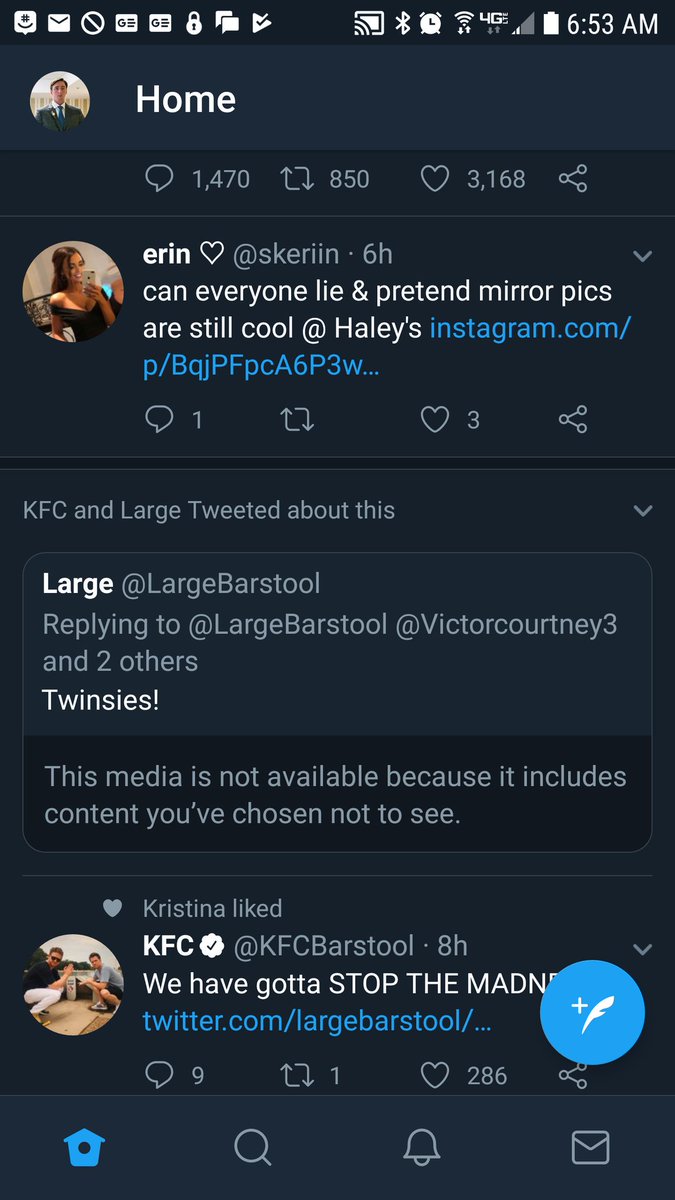Screenshot of a smartphone depicting the home screen with an all-black background. The time displayed is 6:53 a.m., and various indicators show active functions: casting option, Bluetooth availability, and an active alarm. The battery is fully charged, though the signal strength displays few bars. 

At the top, the user’s avatar icon is visible, and the screen shows a Twitter feed thread featuring a tweet from Aaron (@S Kieran) posted six hours ago: "Can everyone line pretend mirror pics are still cool?" replying to @Haley's Instagram-related content. 

A response from KFC Enlarge (@Large Barstool) reads, "Twinsies," followed by a content restriction message: "This media is not available to you because it includes content you’ve chosen not to see." Another user, Christina, responds to KFC with, "We've got to stop the madness." 

At the bottom of the screen are navigation icons for Home, Search, Notifications, and Messaging. A large blue plus symbol with a feather indicates the option to compose a new tweet. It appears that the user has just woken up and is casually browsing through their Twitter feed.